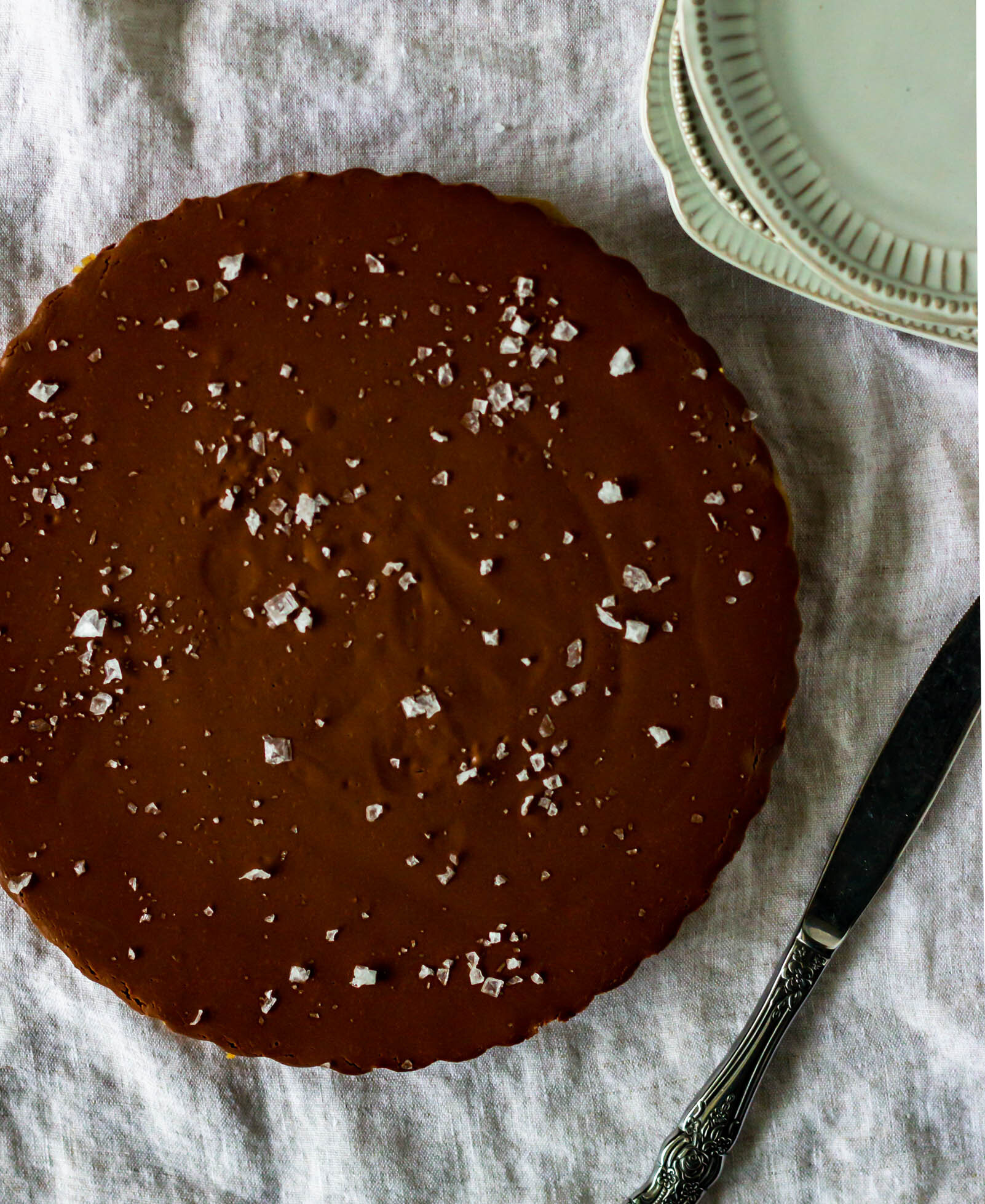The vertically rectangular, full-color photograph, taken indoors under artificial lighting, depicts a staged scene centered around a round, brown dessert that appears to be a cake or possibly a brownie with a chocolate frosting. The cake is generously sprinkled with either sugar crystals or coconut flakes, adding a contrasting white texture on its surface. The setup includes a wrinkled white cloth, potentially cheesecloth or a similar material, covering the entire back and foreground. In the lower right-hand corner, there is a silver butter knife, while the upper right corner features a stack of green serving plates, one of which is round. The setting suggests that dessert is about to be served.